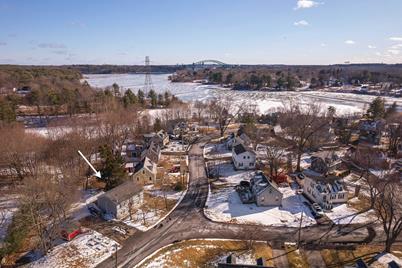The image captures a picturesque, rural residential neighborhood during winter, showcasing a serene landscape dusted with a recent light snowfall. Within the neighborhood, small houses line a Y-shaped road that extends straight before angling off to the right. The terrain is a mix of green grass and patches of snow. In the background, a large steel bridge spans a river, with a cell tower visible on one side. Expansive fields of snow stretch from the residential area to the distant bridge, flanked by dense forested regions on both sides. The trees, bare of leaves due to the winter season, populate the area abundantly, with more trees visible across the river's shoreline. An arrow in the picture points to one of the houses, though its significance is unknown.